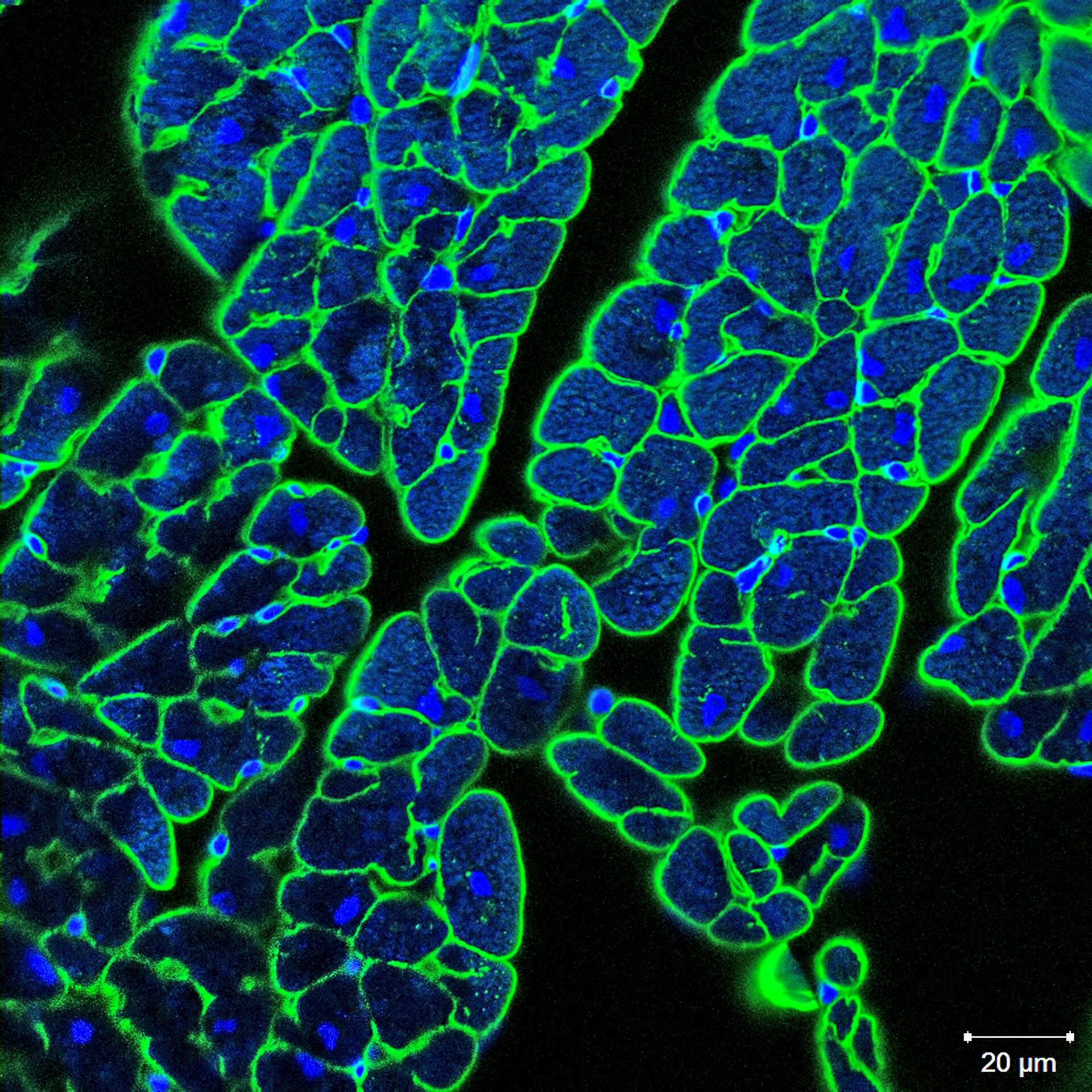The image depicts a microscopic view featuring a black background in the bottom right-hand corner with a measuring guide indicating '20 UM'. The primary subjects in the photo appear as vibrant shapes: neon green outlines with darker blue interiors and lighter blue centers. These colorful shapes are dispersed throughout the image, creating an intricate pattern. The green outlines suggest the cellular walls, while the darker blue interiors represent more structured regions akin to cell nuclei. The overall appearance evokes a leafy pattern with interconnected shapes, possibly resembling leaves viewed at a microscopic scale.